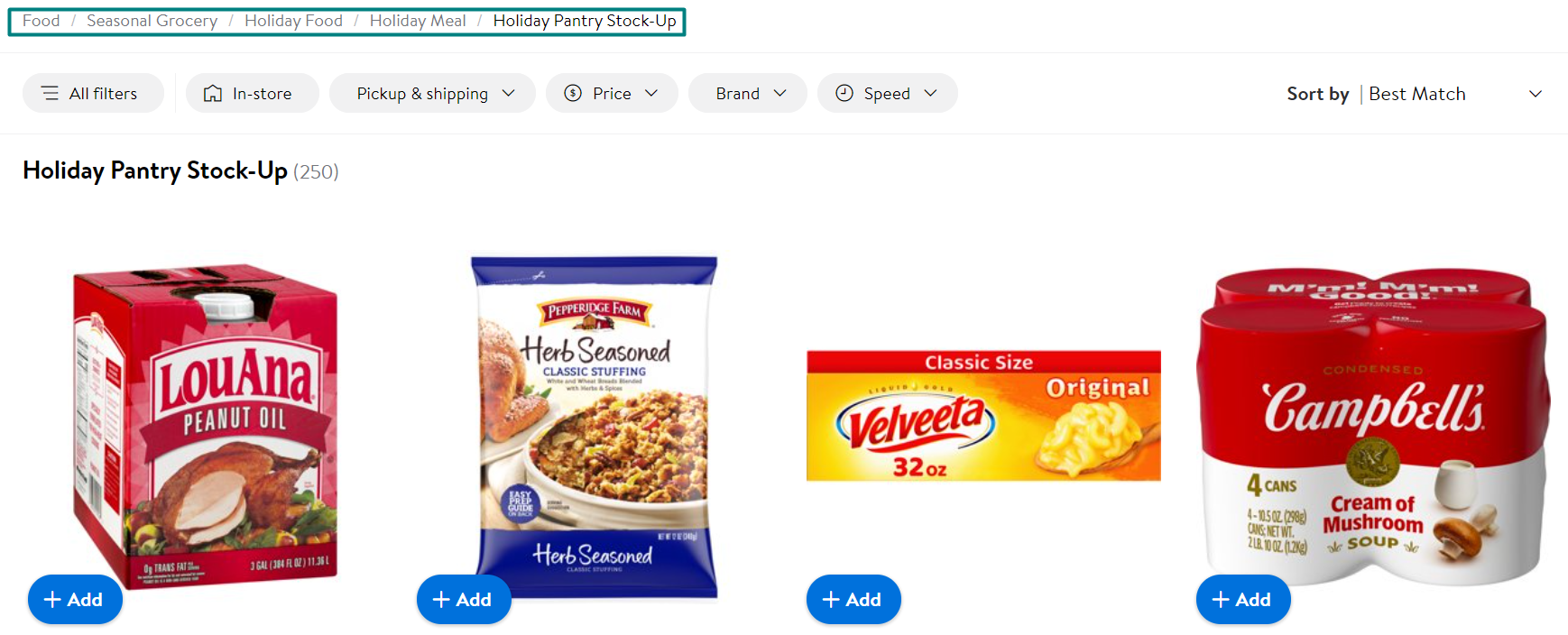The image appears to be a screenshot from a Walmart online store page, specifically within the food section under the seasonal grocery category titled "Holiday Meal." The section features a photo grid displaying four holiday-related grocery items: LouAnna Peanut Oil, Herb-Seasoned Classic Stuffing, a 32-ounce package of Velveeta Original, and a four-can pack of Campbell's Cream of Mushroom Soup. Each item in the grid has a blue "Add" button beside it, but lacks detailed descriptions. The page indicates a total of 250 products available in this subcategory, though only these four items are visible in the image. The products are sorted by "Best Match," and various filters such as "In Store," "Pickup and Shipping," price, brand, and speed options are available for refining search results. Despite the seasonal theme, the direct connection of these items to Christmas isn't immediately clear.